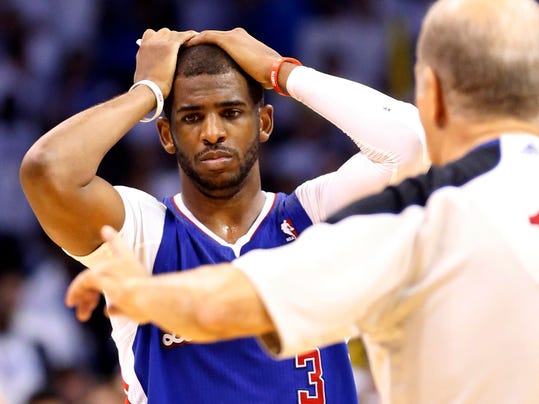The photograph captures a distraught Chris Paul, the NBA player, in a Clippers uniform at the center of the image. He is front and center, with his hands grasping his head in apparent frustration or disbelief. His dark blue jersey prominently displays the number three at the bottom, and the NBA logo is visible beneath his left shoulder. Paul is wearing a long white sleeve on his left arm, accessorized with a red rubber wristband, and a white wristband on his right wrist. To the right side of the image stands an out-of-focus referee, a Caucasian and balding man with gray hair, wearing a white shirt with black shoulder pads. The referee is extending his arm towards Chris Paul, holding out a finger as he does so, possibly indicating a call or foul. The background shows a blurred crowd, hinting at the atmosphere of an indoor, well-lit NBA game. The focal point of the image is clearly on Chris Paul's despondent expression and body language, accentuated by the referee's gesture towards him.